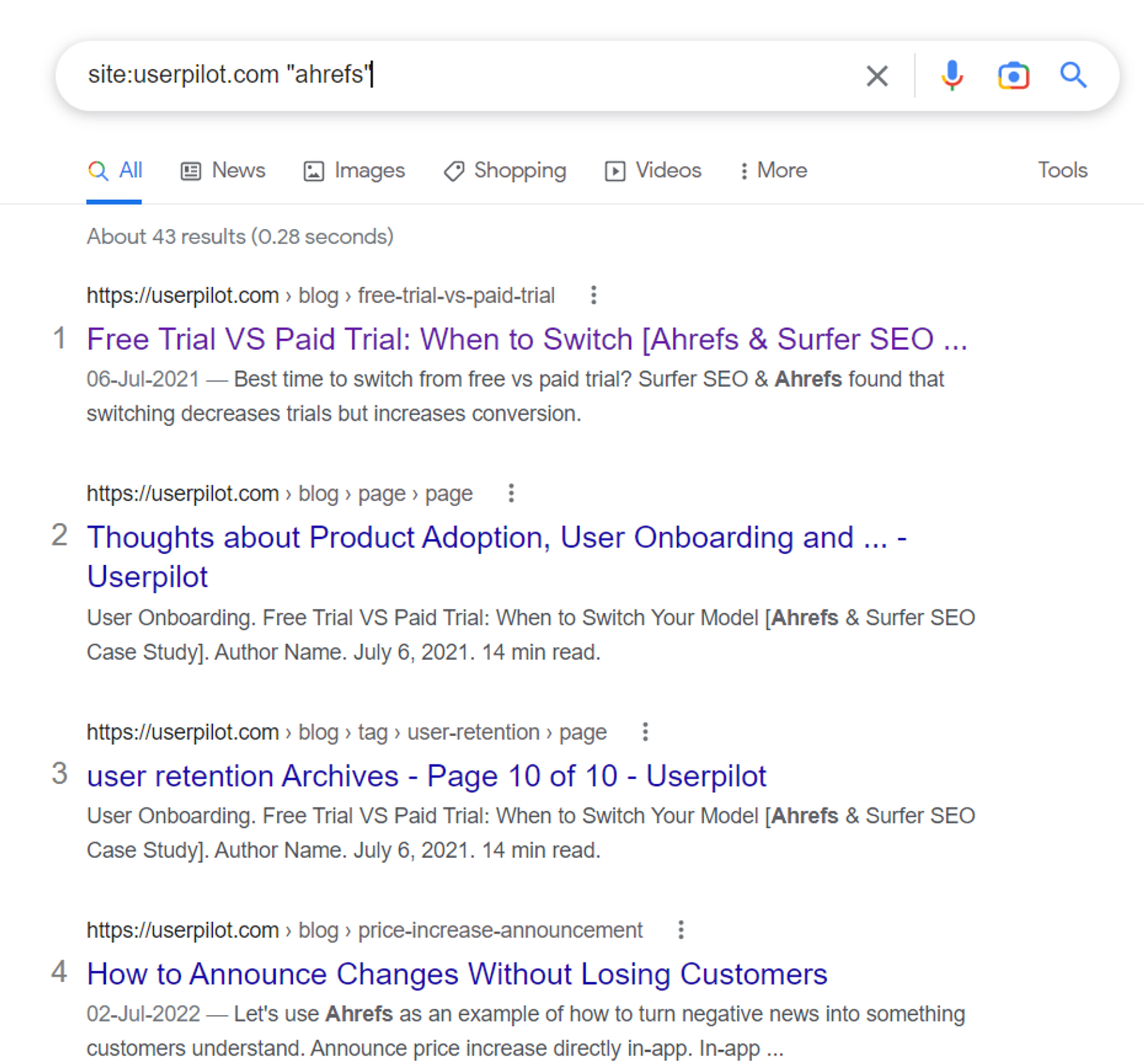This image shows a Google search page where the query `site:userpilot.com (ahrefs)` was entered. The search results are specifically restricted to content from the Userpilot website and include references to "Ahrefs." The top four results are highlighted:

1. **Free Trial vs. Paid Trial: When to Switch | Ahrefs and Surfer SEO**
   - **Brief Description:** This result discusses the optimal time to transition from offering a free trial to a paid trial, incorporating insights from Ahrefs and Surfer SEO.
   - **Caption Underneath:** "Best time to switch from free vs. paid trial?"

2. **Thoughts About Product Adoption, User Onboarding, and Userpilot**
   - **Brief Description:** This piece reflects on various strategies related to product adoption and user onboarding within the Userpilot platform.
   - **Caption Underneath:** "User onboarding, free trial vs. paid trial, when to switch your model, Ahrefs and Surfer SEO case study."

3. **User Retention Archives - Page 10 of 10**
   - **Brief Description:** This entry is part of Userpilot's blog archive, focusing on user retention and onboarding strategies.
   - **Caption Underneath:** "User onboarding, free trial vs. paid trial, when to switch your model, Ahrefs and Surfer SEO case study."

4. **How to Announce Changes Without Losing Customers**
   - **Brief Description:** This article demonstrates how to communicate changes, such as price increases, to customers using Ahrefs as an example for effective in-app announcements.
   - **Caption Underneath:** "Let's use Ahrefs as an example of turning negative news into something customers understand."

These results provide a comprehensive overview of Userpilot's resources on transitioning trials, user onboarding, retention strategies, and customer communication, all through the lens of Ahrefs.